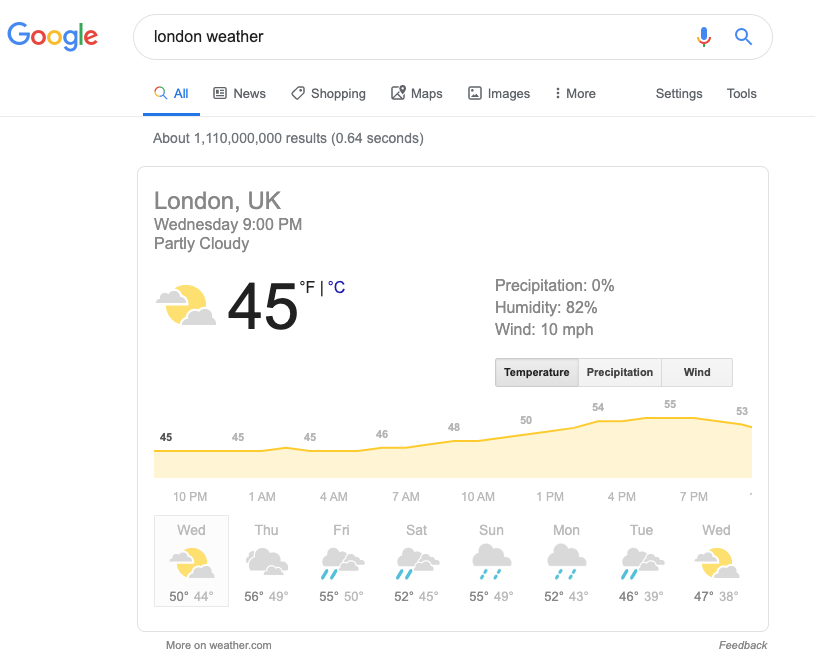Here is the cleaned-up and detailed caption:

---

A computer application graphic provides a weather forecast for London, UK, detailing conditions for Wednesday at 9 p.m. The current temperature is 45°F with partly cloudy skies. Precipitation is at zero percent, humidity is at 82%, and the wind speed is 10 mph. The temperature is projected to remain at 45°F for the next four hours, rising to 46°F by 7 a.m., 48°F by 10 a.m., 50°F by 1 p.m., 54°F by 4 p.m., 55°F by 7 p.m., before settling back to 53°F by 10 p.m. The weekly forecast indicates a high of 50°F and a low of 44°F for Wednesday. Thursday will be cloudy with a high of 56°F and a low of 49°F. Rain is expected from Friday through Tuesday, and partly cloudy skies will return on Wednesday.